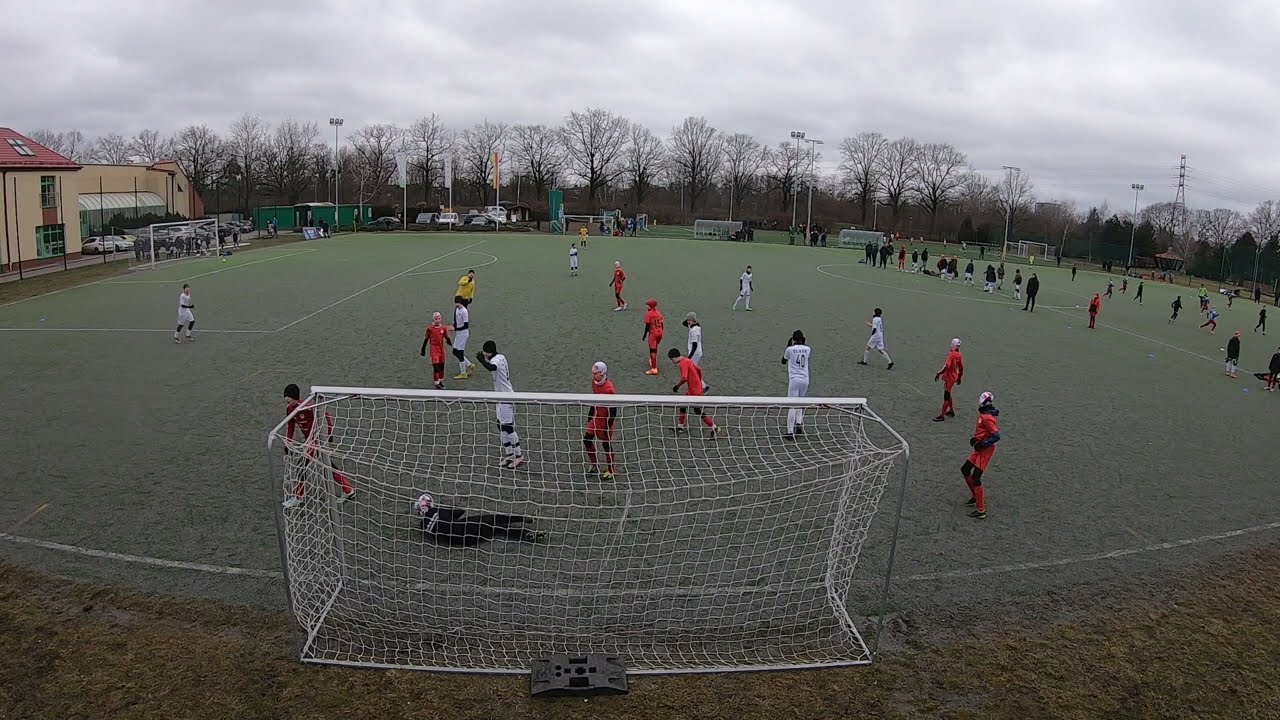This image captures a high school lacrosse game, taking place on a sprawling grass field flanked by multiple net goals. The scene exhibits a large number of players, indicating two games transpiring simultaneously on adjacent fields. The teams are notably wearing distinct uniforms: one in bright orange with black accents, and the other in all white. A notable moment is pictured near the closest goal, where a goalie, dressed in black with a white helmet, has just blocked a shot and is seen sliding on his side. 

Several figures are visible, including a person in yellow, potentially serving as a referee. On the left side of the field lies a substantial tan building with a red roof, possibly a sports complex, underscoring the organized nature of the event. Surrounding the field, a lush expanse of grass leads to a tree-lined horizon, which frames the distant background under an overcast, gray sky.